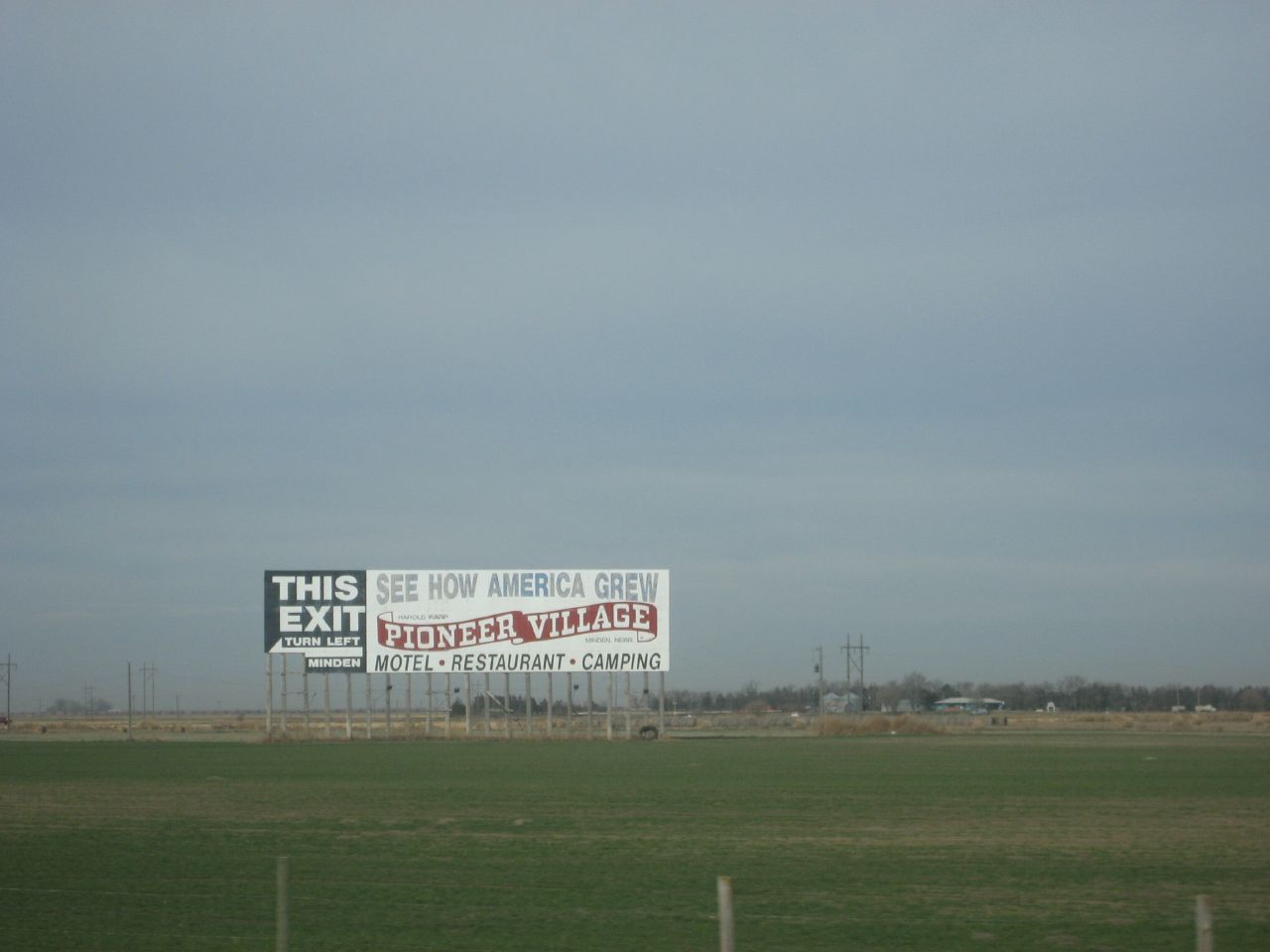In this atmospheric outdoor photograph, the dim lighting casts a serene, almost nostalgic mood over a lush green field, captured in sharp focus. Dominating the scene is a large rectangular billboard in the distance, supported by multiple wooden poles. The sign, visibly worn with a small chunk missing from its lower left corner, directs travelers to "turn left at this exit." Below, it enticingly advertises attractions at a nearby site: "See How America Grew, Pioneer Village, Motel, Restaurant, Camping." In the foreground, a rustic wire fence with sturdy wooden posts adds a touch of rural charm. Beyond the billboard, a scattering of buildings, verdant trees, and intersecting power lines are faintly visible, hinting at a small, quiet community nestled further afield.